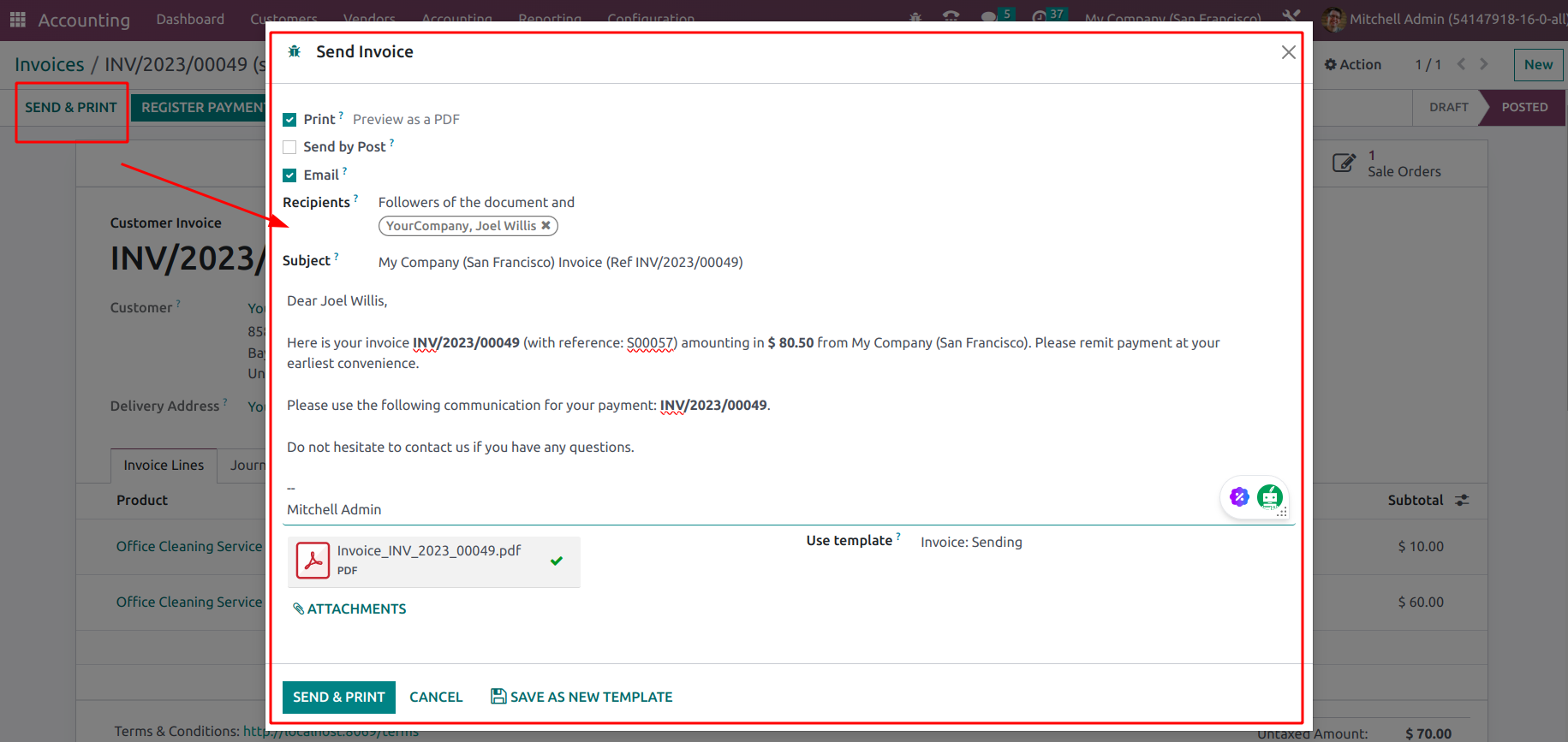**Caption:**

The image is a screenshot from an accounting website. At the center of the screen is a larger rectangular section outlined in red, labeled "Send Invoice." This section is the focal point of the screenshot and details various invoice-related options. Surrounding the main rectangle, the background reveals the rest of the website interface, including sections like "Accounting," "Dashboard," "Invoices," "Send and Print," and "Register Payment" in the top-left corner.

"Send and Print" is also highlighted with a red rectangle, with an arrow directing attention towards the large red-outlined rectangle. Within this primary rectangle, several invoice actions are listed, including "Print," "Preview as PDF," "Send by Post," and "Email," with green checkmarks next to "Print" and "Email."

The next section includes "Recipients," specifying "Followers of the Document" and "Your Company, Joel Willis." The "Subject" line reads "My Company, San Francisco, Invoice Ref INV-2023-00049." Below that, the invoice body starts with "Dear Joel Willis," and continues with a message detailing invoice reference S00057 amounting to $80.50 from My Company in San Francisco. The message requests timely payment and offers contact information for any queries. It is signed by "Mitchell Admin."

An attached PDF titled "Invoice_INV-2023-00049.pdf" is visible below the message. At the bottom, options to "Send and Print," "Cancel," or "Save as New Template" are available for selection.